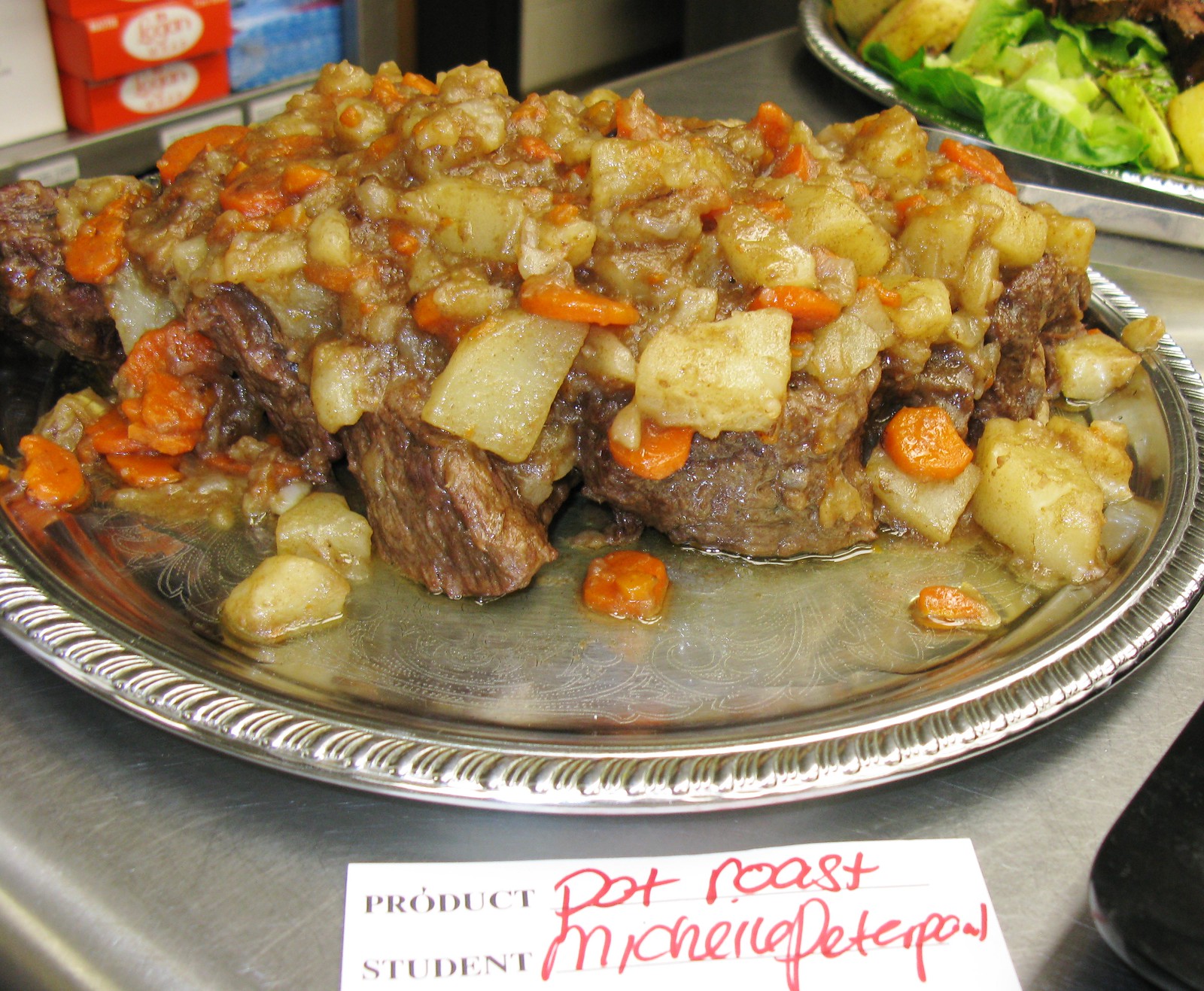In this image, a large platter of pot roast is displayed on a silver restaurant kitchen preparation table. The platter is oval-shaped with ornate edges and contains well-done, juicy beef topped with a generous amount of chopped potatoes and carrots. The dish appears moist and somewhat mushy with a lot of fluid on it. The beef runs the length of the platter, with more potatoes and carrots than meat. 

In front of the platter, a white piece of paper label lies on the table. It reads "Product: Pot Roast" in black typed font with "Pot Roast" handwritten in red marker. Below, it says "Student" in black typed font with the name "Michelle Peterpan" handwritten in black marker, although part of the name appears cut off or smudged.

In the upper right-hand corner of the image, another silver platter is partially visible, containing lettuce and some other food items, one of which appears brown and others yellowish. In the background, towards the left, there are red and blue boxes stacked on a shelf, indicating kitchen supplies.